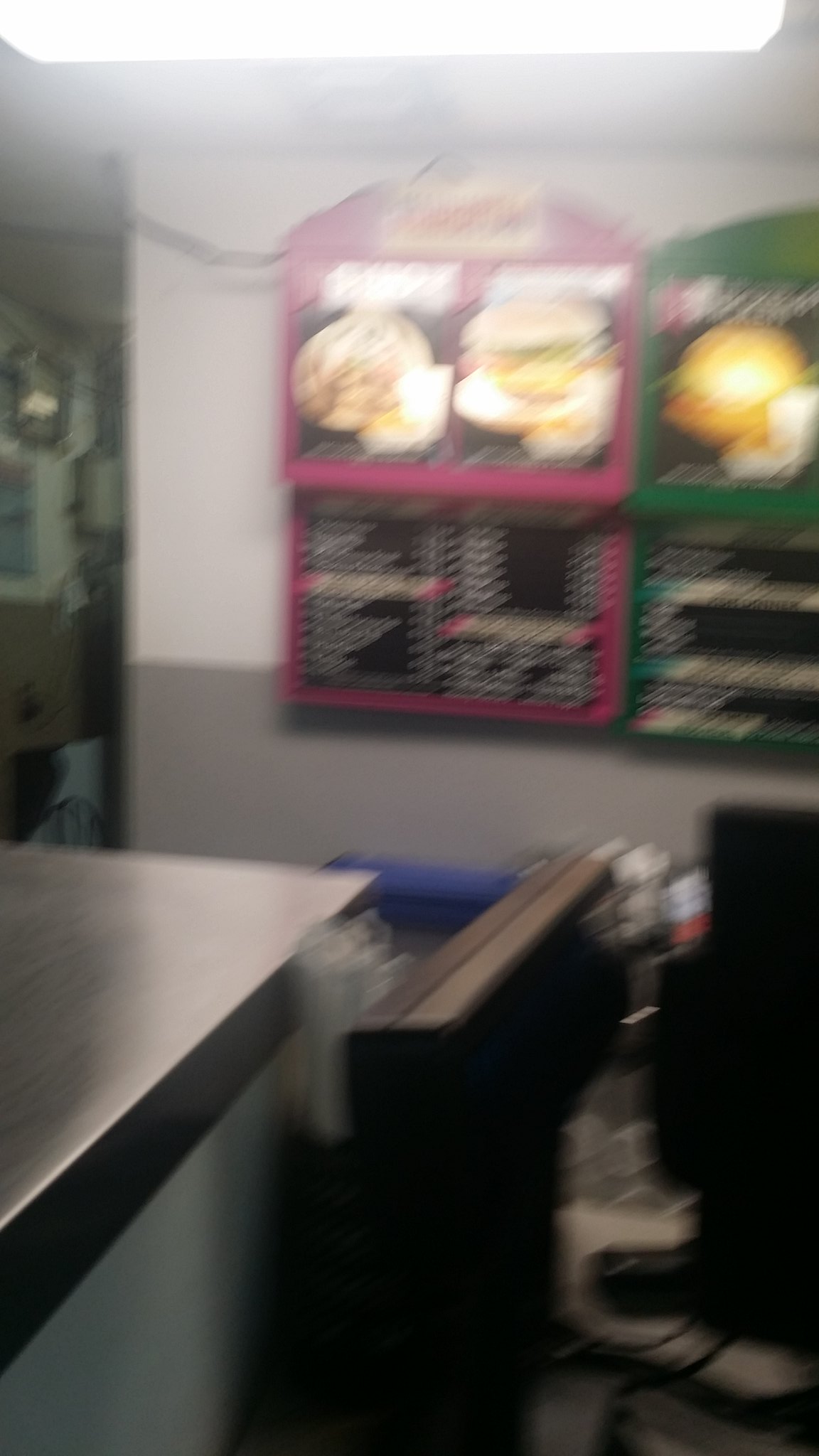A blurry photograph captures the inside of a restaurant. The image, though unclear, appears to show a corner where customers might stand to place their orders. In the background, a wall faces the camera, adorned with two distinct menus side by side. The first menu, predominantly pink, features images at the top that resemble a hamburger and a plate of food positioned next to each other. To the right, extending into the shot, is a green menu which also seems to display a hamburger among its offerings.